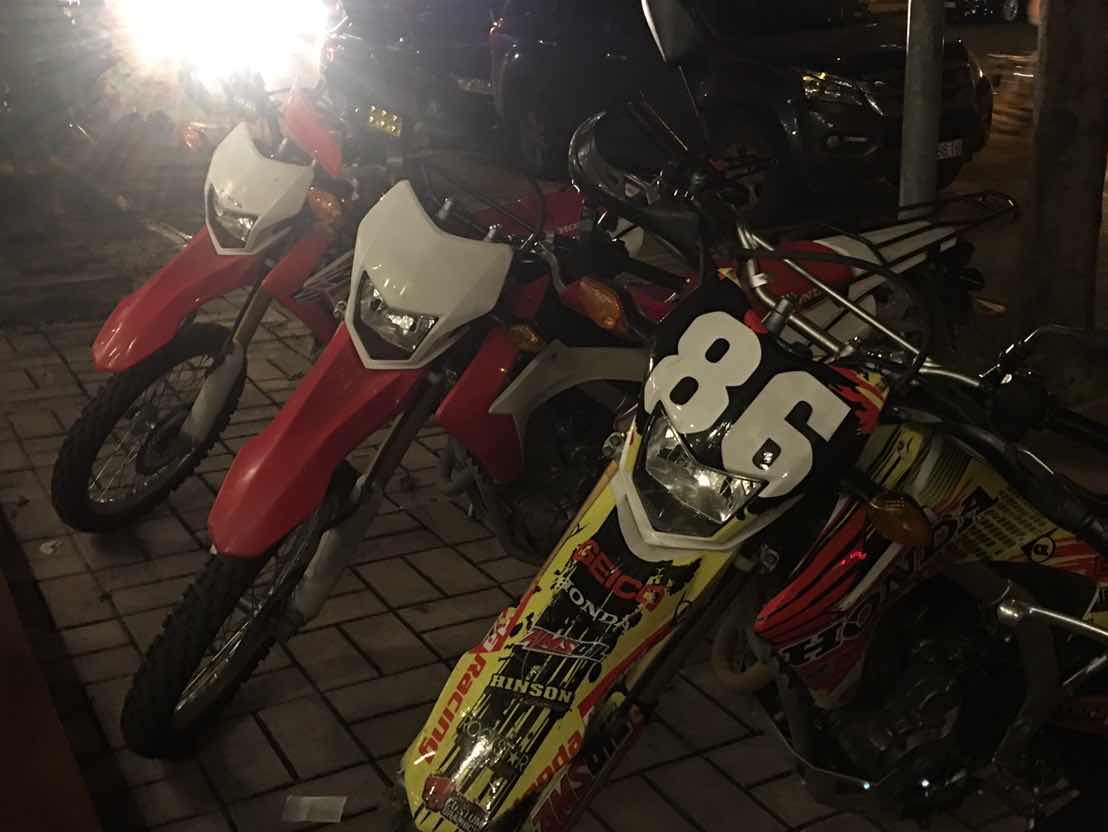In this nighttime outdoor image, three motorcycles are prominently displayed, all parked close together. Two of the bikes have striking red and white color schemes and appear to be of the same make, possibly motorbikes or mountain bikes, though the front wheels make this somewhat uncertain. The third bike, on the right-hand side, stands out with multiple sponsor decals, including the number 86 and names such as Honda, Hinson, and Geico, suggesting it's a racing bike. The scene is somewhat obscured by a strange light in the upper left corner, making it hard to discern finer details. Additionally, there are cars parked behind the bikes, and a tire is visible on the right.